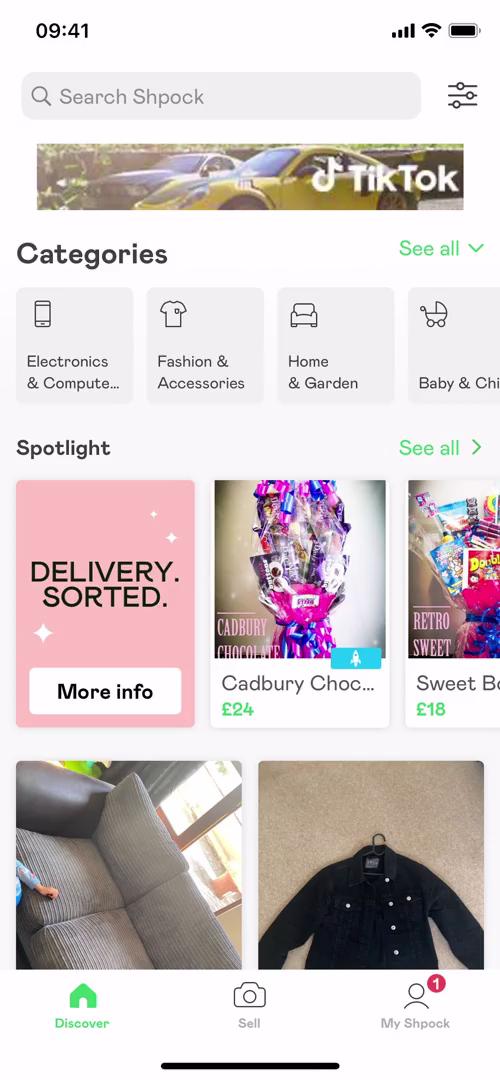The image is a screenshot from a mobile phone, depicting an app interface with a white background. In the status bar at the top, it shows the time as 09:41, followed by indicators for strong cellular signal (four bars in black), a Wi-Fi connection, and a fully charged battery. Below the status bar, there is a gray search bar with "search SHPOCK" typed into it.

The main part of the screen is divided into several sections. The first section features a long, skinny rectangular image of a gray and yellow car. To the right of this image is the word "TikTok" accompanied by a music note icon.

Further down, the interface presents a categories section. "Categories" is written in the top left corner with "See all" in green on the right, accompanied by a dropdown arrow. There are four gray squares underneath this section labeled "Electronics and Computer," "Fashion Accessories," "Home and Garden," and "Babies and Children."

Below the categories section, there is a "Spotlight" section with "See all" in green on the right. This section contains three square images. The first image is pink and has the text "Delivery Sorted" with a white "More Information" button. The second image appears to feature "Cadbury chocolate," displayed alongside pink and blue ribbons. The third image seems to showcase retro sweet chocolate.

At the bottom of the screen, there are two more rectangular images. One displays a gray couch, and the other shows a black jacket.